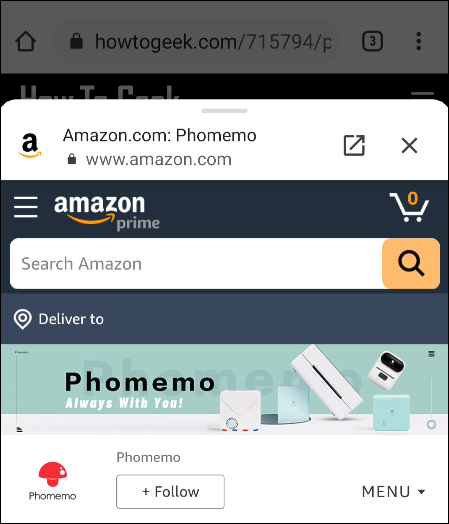This is a detailed screenshot featuring a white background. The screenshot displays the URL "howtogeek.com/7157794/p" and "amazon.com/FOMEMO." Additionally, the Amazon homepage URL "www.amazon.com" is visible. The interface includes a hamburger icon, signifying the menu, and an "Amazon Prime" indicator. There is also a shopping cart icon showing zero items. A prominent search box with an orange square and a black magnifying glass is present.

The main content highlights the brand "FOMEMO" multiple times, including a tagline that reads "FOMEMO Always With You." An image of FOMEMO with a red mushroom design is featured. Below is a black rectangle with a "Plus Follow" button. A "MENU" option in uppercase letters accompanied by a down arrow is also visible, suggesting a dropdown option.